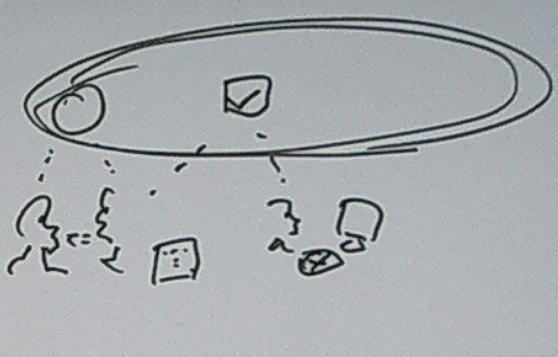The artwork is a monochromatic black-and-gray piece with a gray background. Dominating the composition is a large black oval extending horizontally across the canvas. Within this oval lies an encompassing circle, filled with intricate black line work and symbols. 

To the far left, close to the border, a circle with a central line intriguingly resembles a heart or a tomato. Adjacent to this, a prominent box with a bold black checkmark sits in the middle of the scene, outlined distinctively in black. Radiating from this central box are various elements, including a series of black marks that contour the profile of a face. 

Further along, another black mark appears, leading to a small black box containing an X, while directly above it is a square with a hook-like extension. On the leftmost side, another line stems from the central box, connecting to yet another outlined box. 

Beneath the heart- or tomato-like circle is a figurine suggestive of a right-side facial profile, featuring a sharply pointed head, a prominent nose, and a neck area that abruptly ends in a cutoff. Additionally, the lower part of the artwork includes a small letter "C," followed by an equal sign, and two small squiggly lines stacked vertically, adding to the piece's detailed complexity.